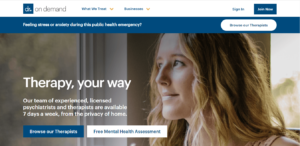A small screenshot depicts a therapy website. At the top, there's a white banner with partially legible text, seeming to say "On Demand." Adjacent to this are two drop-down menus, along with "Sign In" and "Login" buttons on the right side. Beneath this is a blue banner featuring white text and a white button on the far right, though the specifics of the text are unclear.

The main area of the screenshot showcases a large rectangular image of a Caucasian blonde woman gazing out a window to the left. Superimposed on this image is the prominent text "Therapy Your Way" followed by a paragraph: "Our team of experienced, licensed psychiatrists and therapists are available seven days a week from the privacy of your home." Below this are two buttons—one blue and one white, each containing text that is illegible due to the screenshot’s small size.

Overall, the screenshot clearly illustrates a user-friendly interface for a therapy website that offers remote therapy sessions via video chat, despite the difficulty in reading finer details.